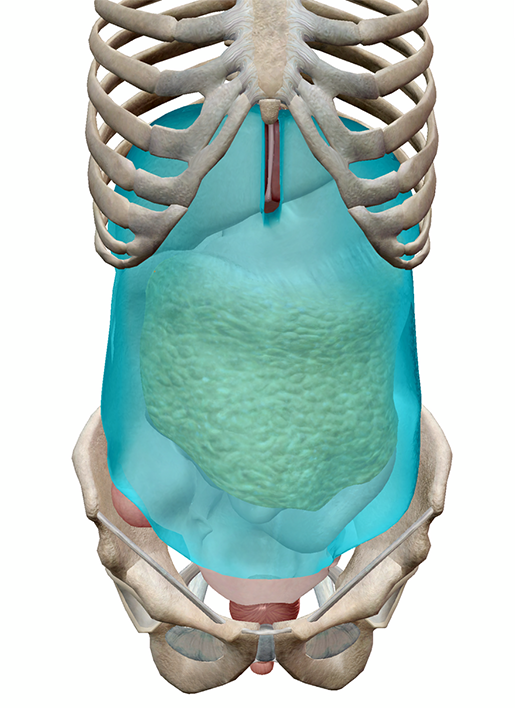This digital rendering presents a detailed, cartoon-style 3D model of the human torso extending down to the pelvis. The image features a white skeletal structure, including the ribcage and pelvic bones. Over the internal organs in the abdominal area, there is a blue translucent highlighting that appears to represent adipose tissue, or body fat. This blue highlighting obscures the actual organs, but some details still peek through. The yellowish regions represent fat deposits, while the internal organs show varying shades of pink and red. Notably, a red line runs vertically from the center of the ribcage down toward the blue-highlighted area. The background of the image is stark white, devoid of any additional elements, placing full emphasis on the anatomical structures.